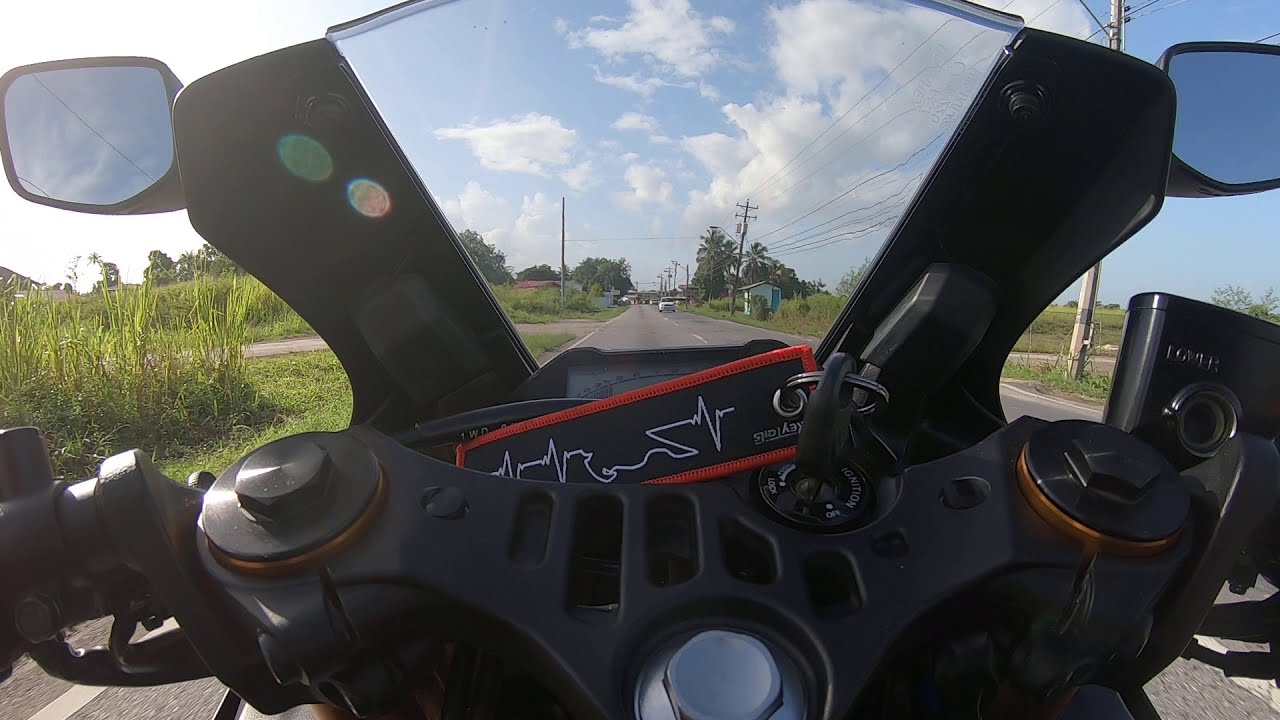The image captures a point-of-view (POV) shot from someone riding a state-of-the-art, black motorcycle. The rider, whose hands are not visible, is traveling on a two-way concrete highway. The perspective shows the motorcycle's dashboard, ignition with a black keychain featuring a red border and white heartbeat pattern, and rear-view mirrors atop the windshield. The road stretches ahead into a partly cloudy blue sky, with the rider positioned in the left lane, hinting at a location outside of America. Oncoming cars appear on the right-hand side lane, while electrical poles with wiring line the right side of the road. Surrounding the highway are expanses of grass and bushy stretches of land, evoking a rural, open-field landscape with minimal housing or structures visible. There’s a distant parallel street to the left, but it hasn’t been reached yet. Electrical poles with wires can be seen to the right, and the overall scene feels like a journey through farmland or pastoral countryside.